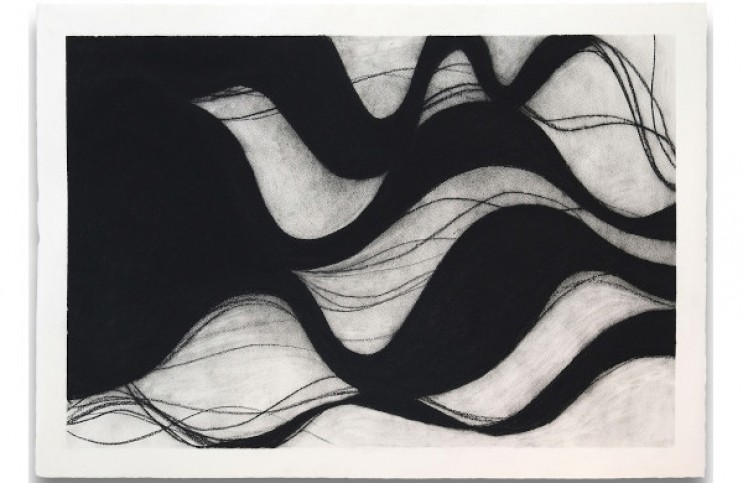This black and white photograph features an intricate design of wavy black lines against a grayish-white background. The canvas, bordered by a crisp white frame, is dominated on the left side by a dense, solid cluster of black lines, which resemble strands of hair, yarn, or twine. These lines are uneven and heavily smudged, creating a sense of chaotic density. As they move towards the right side of the image, the lines thin out into more delicate, singular strands that mimic the larger curves. The more substantial waves and curves on the left peter out towards the right, creating a gradient of density and complexity. The top portion of the image shows heavier, more pronounced smudging compared to the bottom, adding to the textured, almost tangible quality of the artwork.